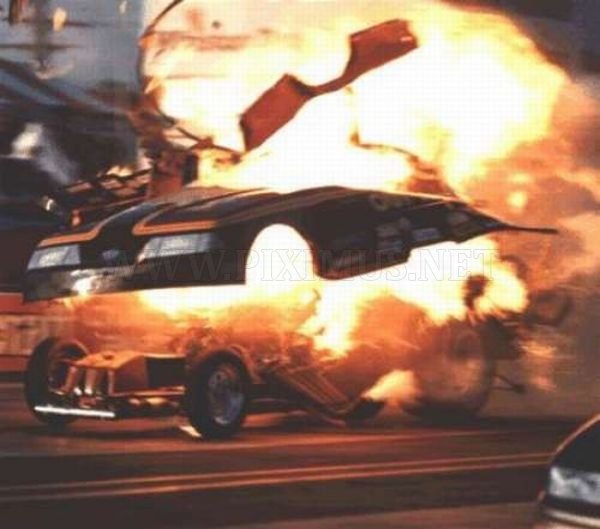The image captures an intense car explosion at night, presenting a dramatic and chaotic scene. The main focus is a car in the midst of a fiery combustion, with its hood and upper frame catapulted upwards from the intense blast. The vehicle's wheels remain grounded, still touching the road beneath, which is dimly visible in the otherwise dark environment. The explosion emanates a powerful fireball with shades of red, orange, yellow, and white flames, engulfing the car from top to bottom and extending upward, covering a significant portion of the frame.

The photograph seems zoomed in, emphasizing the exploding car while the surrounding area remains largely obscure and dark. There is debris and shrapnel suspended in the air above the car, pointing to the violence of the blast. In the lower right corner of the image, a faint headlight of another car is visible, suggesting the presence of a nearby vehicle. Additionally, there are hints of buildings in the background, partly illuminated by the explosion. The framing of the image shows the car from a front and side angle, revealing that the vehicle appears to be black, possibly with some orange striping. The composition, lighting, and visible elements make the scene reminiscent of a dramatic still from an action movie.